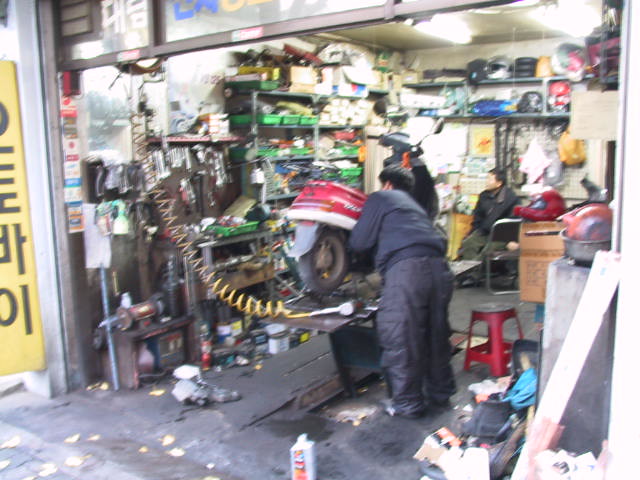The image showcases a cluttered, makeshift garage or workshop, likely an automotive repair shop. The ground is dirty and scattered with debris, including rags, tools, and other miscellaneous items. At the center, a man dressed in a navy blue jacket and matching thick cargo pants is working on a red and white scooter, possibly inflating the tires with an air compressor, identifiable by its coiled yellow cord. The scooter is precariously placed on a shelf rather than a proper lift. The workshop is crowded with various objects: red and pink bike helmets on shelves, green bins overflowing with items, and a red stool. In the blurred background, another man dressed in black, with black hair, is sitting and gazing off to the left. Korean script is visible on the left side, adding to the impression of an eclectic, busy environment filled with small objects and clutter.